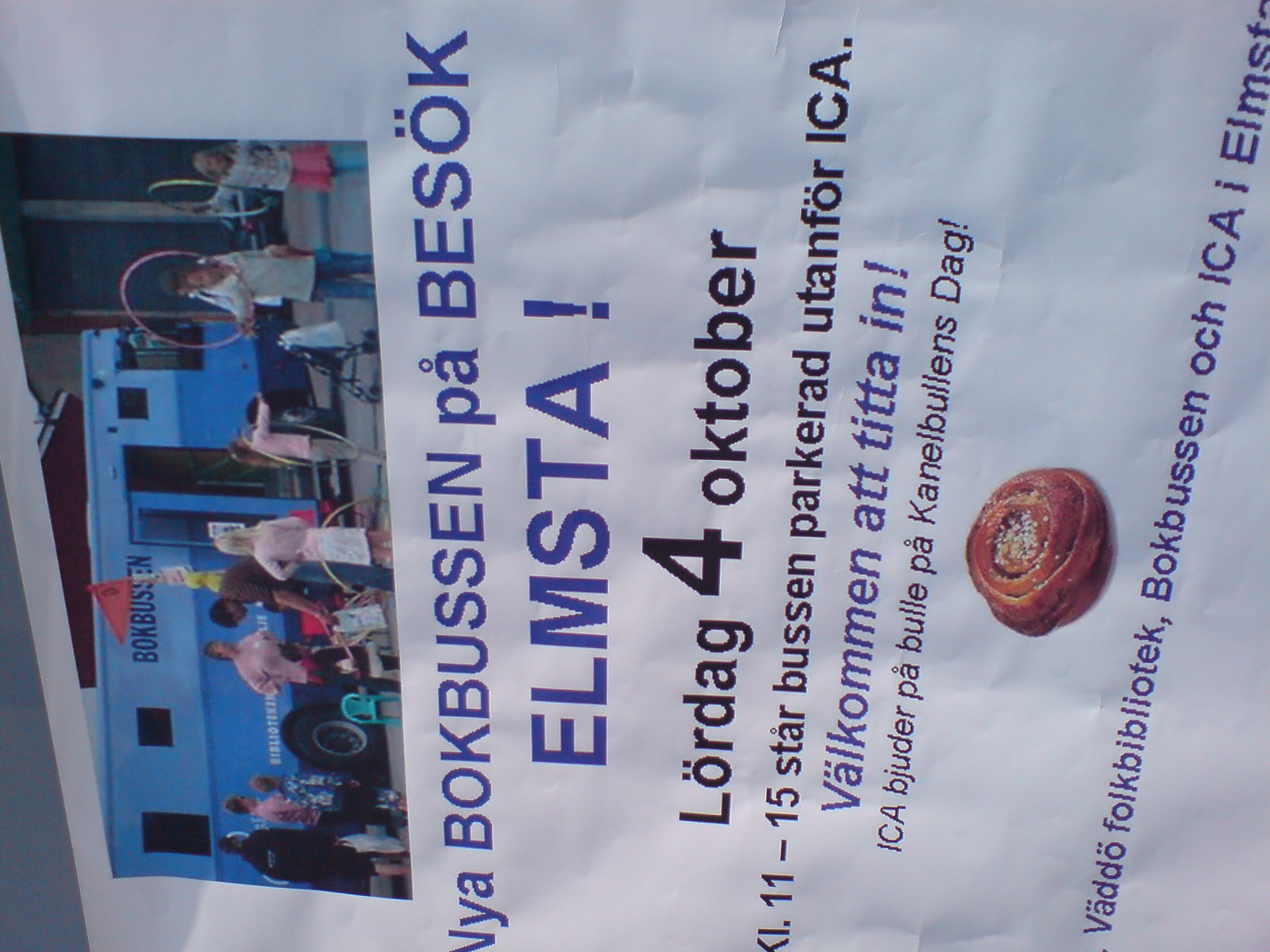The image is a sideways advertisement printed on white paper that appears crinkled and old. The text is in German, comprising both blue and black fonts. At the top of the advertisement, there is a photograph featuring a light blue and dark blue bus or van with a group of people, including children holding hula hoops and someone with a stroller, standing in front of it. The people are dressed in various colors like red, white, pink, yellow, turquoise, black, and white, adding a festive atmosphere. A triangular red flag can be seen in the scene. To the right side of the poster, there is an image of a round, brown pastry with white speckles, possibly pearl sugar, that resembles a Danish.